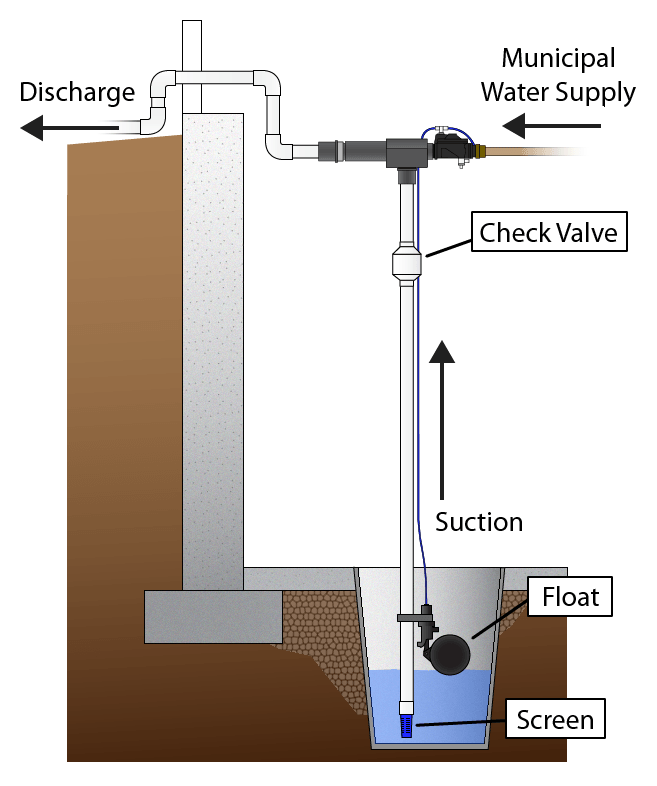This diagram illustrates the workings of a water supply system, potentially for a municipal setup or similar application. The background of the image is white, offering contrast to the detailed components depicted. On the left-hand side, a gray pipe is labeled "Discharge" with an arrow indicating leftward flow. This pipe runs horizontally across the top of the diagram and overlaps with another pipe, which is labeled "Municipal Water Supply," also pointing left.

Between these two main pipes, a vertical white pipe extends downwards and is marked with a box labeled "Check Valve." Below this, the pipe continues into a section filled halfway with water, depicted in a basin embedded within a brown-colored area, signifying dirt or earth. At the bottom end of the pipe submerged in water, there is a blue tip labeled "Screen," with an arrow labeled "Suction" pointing upwards towards the check valve.

Adjacent to the blue tip, a black ball labeled "Float" is shown, and a black wire is connected to it, indicating its attachment to the piping system. The diagram highlights the flow path and key components such as the screen, float, suction, and check valve, providing a comprehensive overview of the water supply system encased within the brown earth-like area.